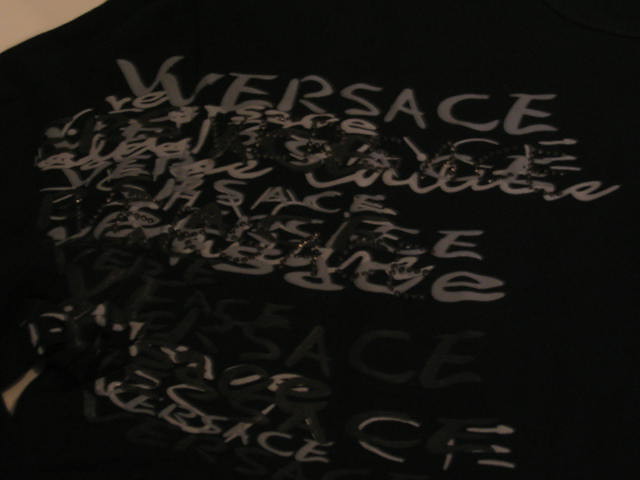The image appears to be a photograph of a black t-shirt featuring a design that mimics high-end fashion brand merchandise. The design prominently displays the word "V-V-E-R-S-A-C-H-E," a deliberate misspelling of "VERSACE," likely suggesting a knockoff or parody of the original brand. The text is repeated in various colors and scripts, creating a layered and chaotic visual effect reminiscent of Jackson Pollock's abstract expressionist paintings, though achieved with text rather than paint. The colors of the text include shades of gray, white, and dark gray, contributing to a somewhat muddled and illegible overall appearance. The image itself is dimly lit, seemingly taken without a flash, which further obscures the details and enhances the grungy, counterfeit aesthetic of the t-shirt.